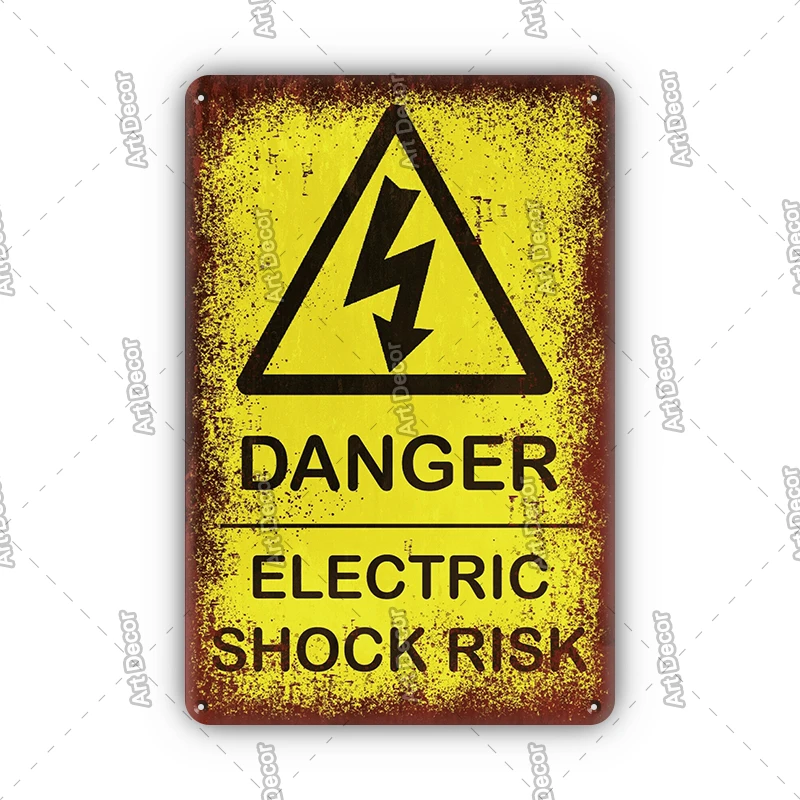The image showcases a vintage-style, yellow danger sign with a rusted appearance, likely intended for decorative purposes in a bedroom or man cave. The sign prominently displays a black-outlined triangle at the top, within which is a black lightning bolt with an arrow, symbolizing the risk of electric shock. The text on the sign reads "Danger" at the top, followed by a separating line, and then "Electric Shock Risk" beneath it. The design includes four small holes in the corners for easy mounting. The sign's aged look is enhanced by rust details, though it is believed to be deliberately painted to appear old, rather than genuinely rusted. Additionally, there are multiple "Art Decor" watermarks surrounding the sign, indicating its protected status and decorative use.